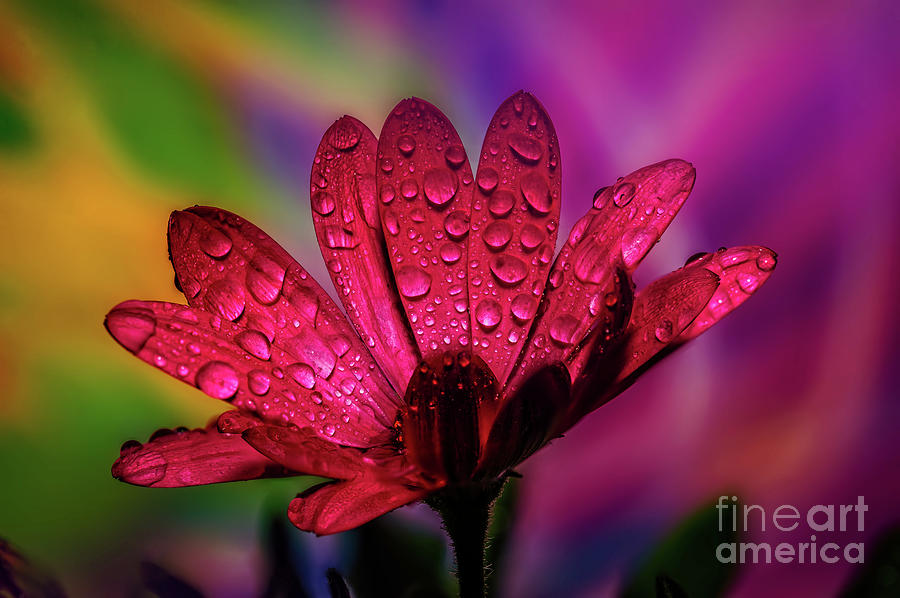The image is a close-up of a vibrant pink daisy, with petals that hint at a touch of red and are adorned with delicate raindrops, suggesting a recent rain. The flower’s long, fine petals resemble the shape of a handheld fan and are slightly pointed upwards but not fully extended. The underside of the flower shows green leaves holding it in place with a faintly fuzzy green stem extending from the bottom. The background is a computer-generated blur of colors; the right-hand side is bright pink, the middle features varying shades of purple, green, and yellow, and the left side blends green and yellow hues. The blurred, undefined colors create an abstract backdrop, making the daisy stand out prominently. In the bottom right-hand corner, the words “Fine Art America” are visible.